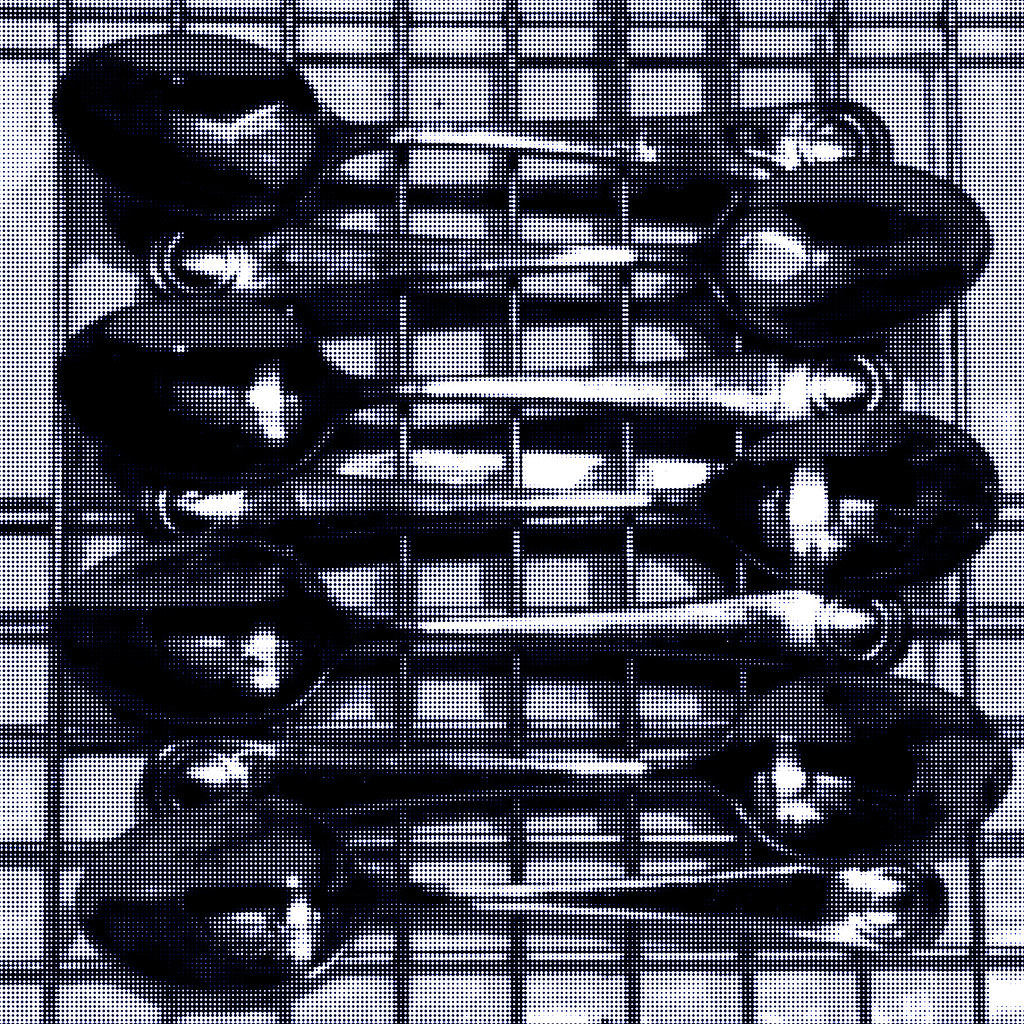This grayscale image features seven silver spoons laid out on a metal rack, resembling a cooling rack for cookies. Each spoon is meticulously arranged in alternating directions: starting with the first spoon pointing left, the second right, continuing this pattern up to the seventh spoon. All of the spoons are positioned upside down with their bowls resting on the rack, reflecting light and casting subtle shadows on the crossbars. These spoons have wide handles, each adorned with a distinctive design comprising a smaller circle within a larger one at the base. The high-contrast black and white filter gives the spoons a somewhat surreal, almost animated look. Below the spoons, a small, square-like texture of the metal surface is visible against a light gray background.